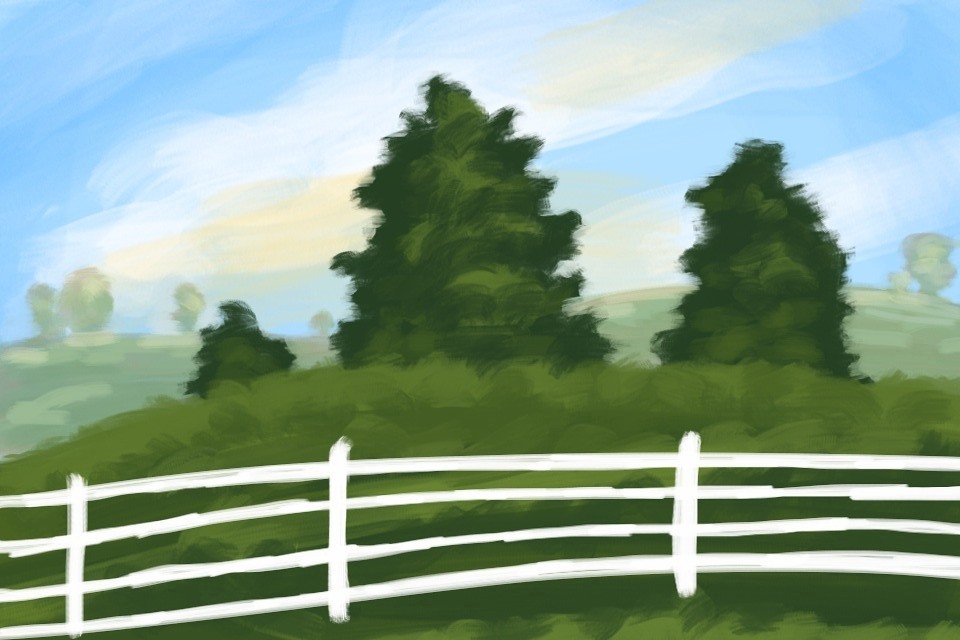The image showcases a rudimentary, somewhat blurry painting of a serene landscape. Dominating the foreground is a white picket fence, stretched from left to right, featuring three upright posts and four uneven, jagged rails. Beyond the fence, lush green hills roll gently, with a mixture of dark and light green hues illustrating dense foliage. Towering evergreens, depicted with a shaggy and lumpy appearance, punctuate the hill's landscape. The clear blue sky above is streaked with white clouds that form diagonal patterns, interspersed with traces of orange and yellow hues adding a warm glow to the scene. Contrasting the main foreground hill, where three evergreens stand prominently, the background features additional scattered trees that recede into the horizon. The overall effect is a jumbled yet vivid representation of nature.